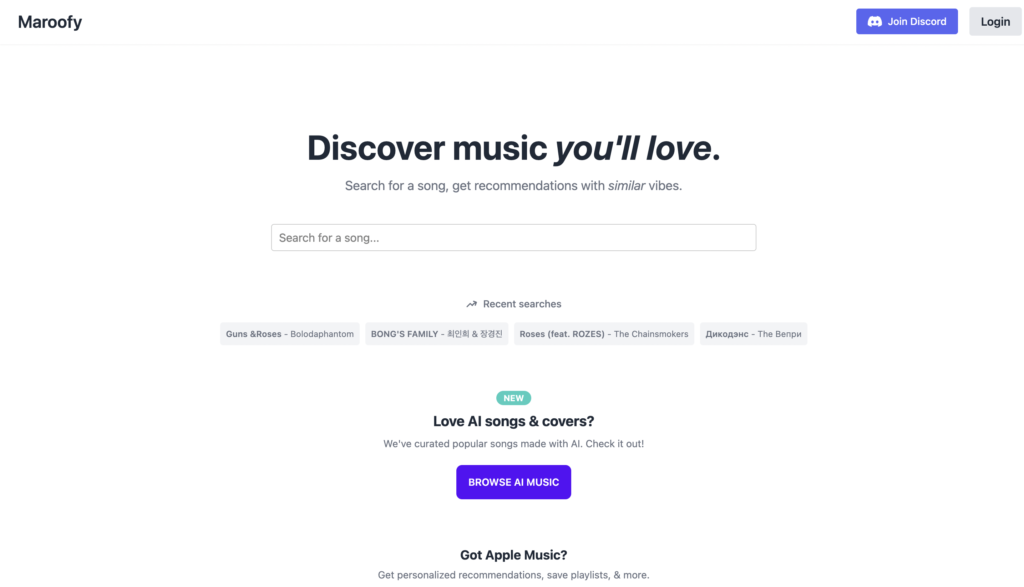Screenshot of the Maroofie website homepage showcasing its music discovery features. In the center of the screen, a prominent banner reads "Discover music you'll love." At the top right corner, there are two buttons: a blue button labeled "Join Discord" accompanied by the Discord logo, and a gray button labeled "Login." 

Below the main banner, there is a search prompt instructing users to "Search for a song, get recommendations with similar vibes," followed by a text box with placeholder text saying "Search for a song." 

Further down, under the heading "Recent Searches," the site displays a list of recently searched songs including "Roses" featuring Roses by The Chainsmokers and two songs in different languages. 

Towards the bottom of the page, a section titled "Love A.I. songs and covers" highlights curated popular songs made with A.I. technology. A blue button at the bottom invites users to "Browse A.I. music."